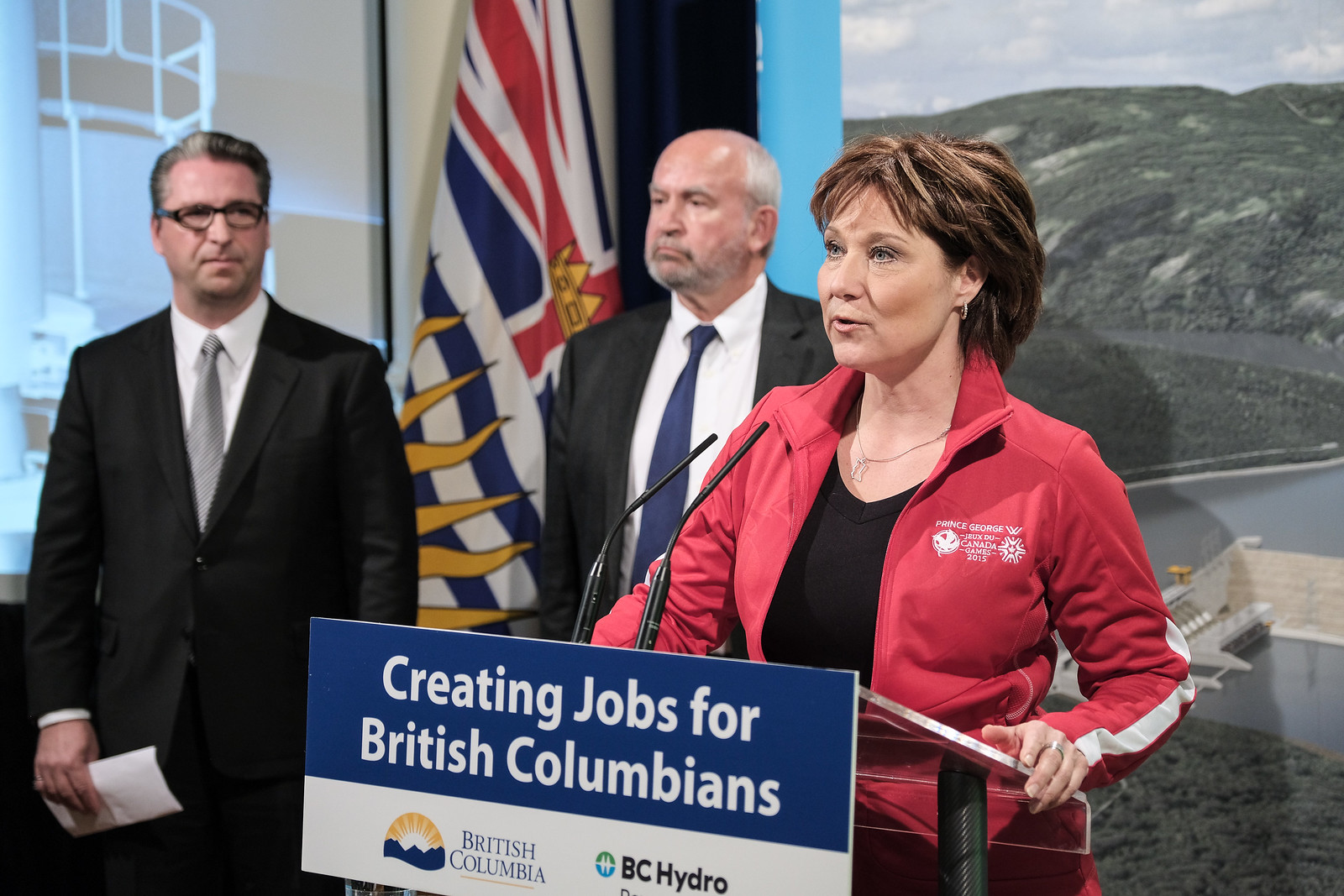In the image, a woman in her early 50s is speaking at a podium during a political event. She is wearing a red zip-up sweatshirt with a white stripe on the sleeve and the text "Prince George Canada Games 2015" on the chest, paired with a black V-neck shirt and a gold necklace. She has short brown hair that falls slightly past her neck and wears gold earrings. The podium is adorned with a sign that reads "Creating Jobs for British Columbians," accompanied by the logos for British Columbia and BC Hydro. Two men stand behind her, facing the crowd. To her right is an older man with white hair, dressed in a black suit, white collared shirt, and navy tie. To her left stands another man with gray hair and glasses, wearing a black suit and gray tie. A flag featuring blue, red, and yellow stripes is positioned between the two men. The background includes a large image depicting hills and sky, suggesting a scenic outdoor view, and a presentation screen is visible behind the gray-haired man.